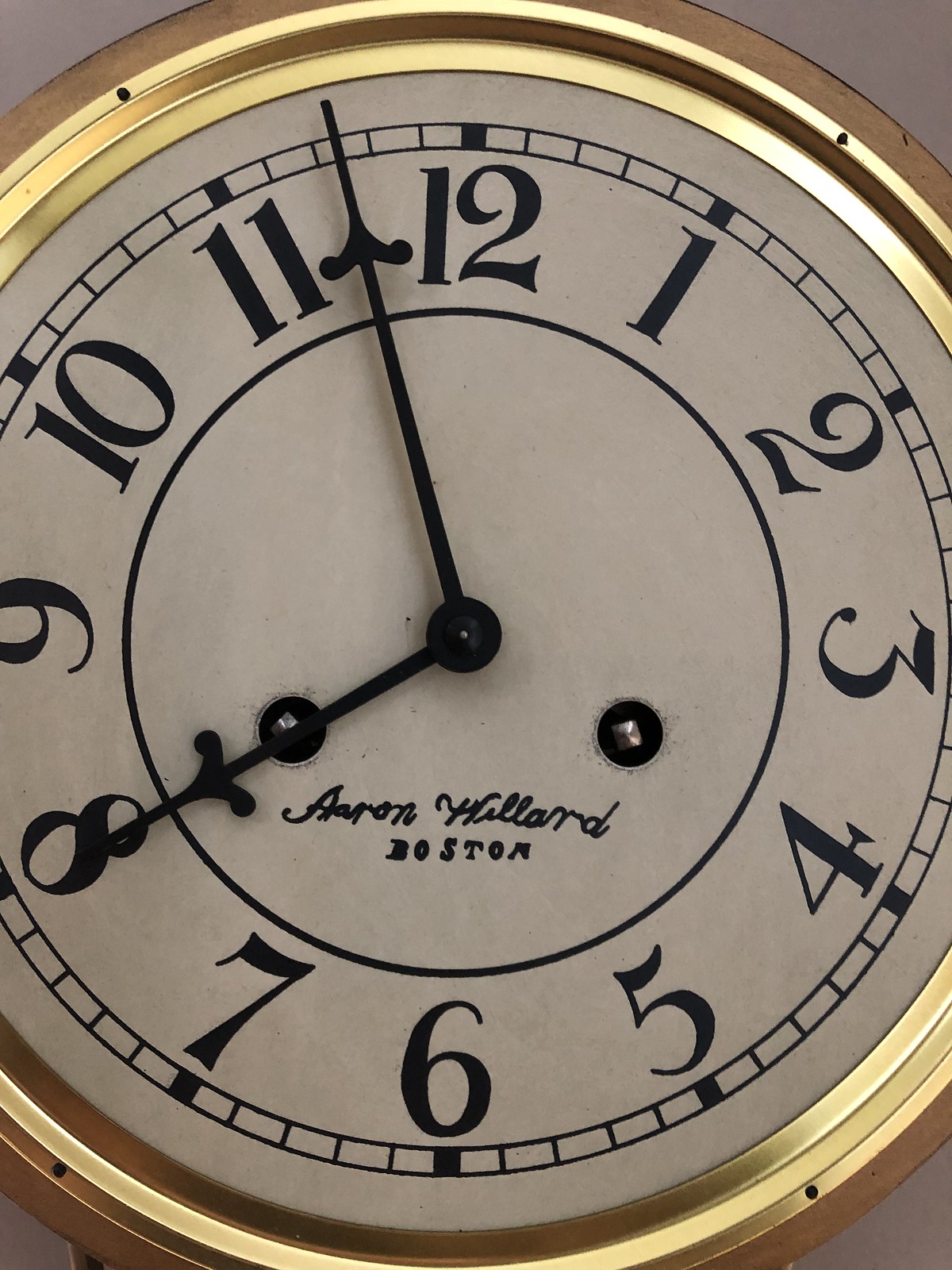A classical timepiece branded "Aaron Hillard, Boston" is showcased, likely a wristwatch rather than a wall clock. It features elegant Breguet-style numerals from 1 to 12, set against an off-white background. The minute hand is notably longer than the hour hand, both in a subtle black hue. The watch is encased in a refined yellow gold enclosure, resting delicately on an off-white table that exhibits a faint pinkish hue.